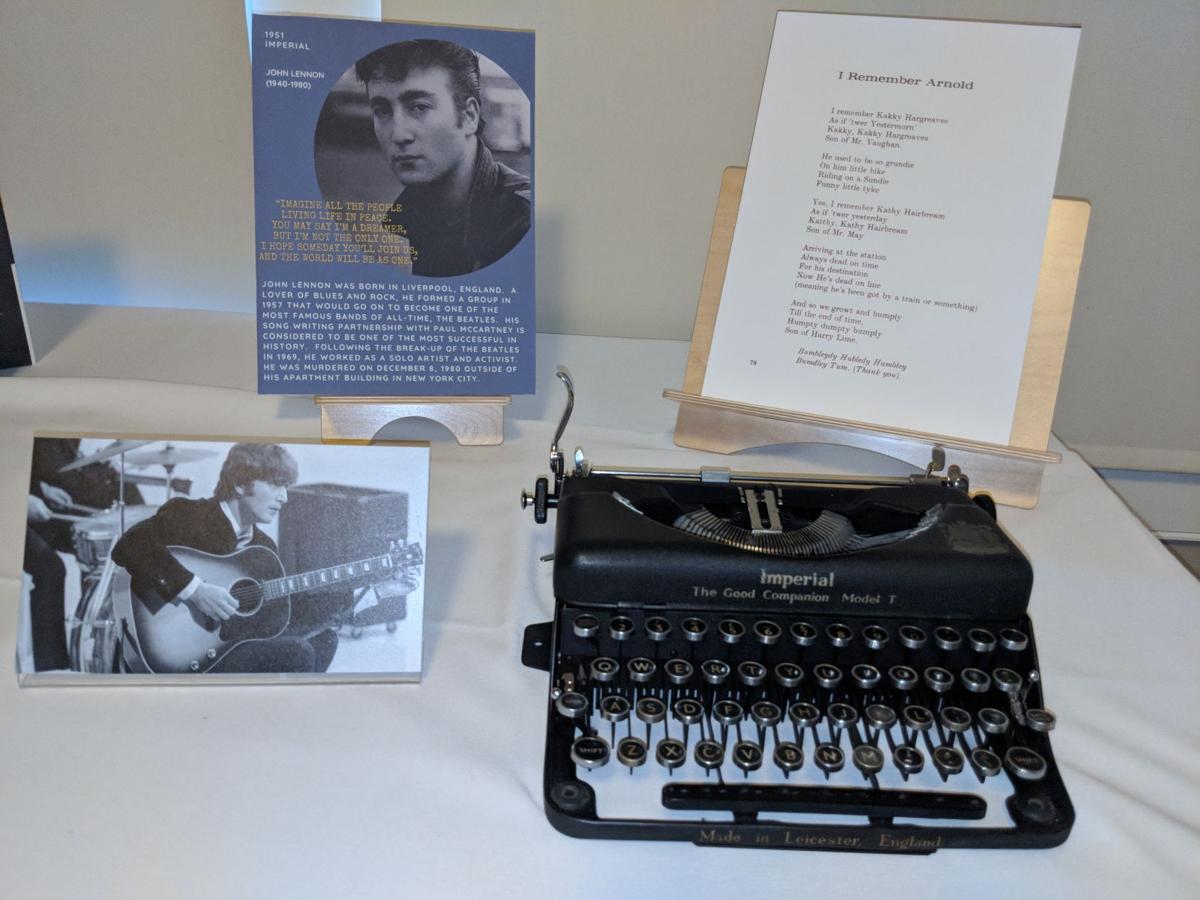The image depicts an indoor museum display dedicated to John Lennon. Central to the display is a poster board featuring Lennon's biography and notable quotes, adorned with a circular image of him at the top, with the heading "1951 Imperial" and the timeline "John Lennon 1940 to 1980." Below this are a photograph of Lennon playing a guitar on stage, with drummers and cymbals visible in the background, and a typed song titled "I Remember Arnold" perched on a pedestal in the upper right-hand corner of the table. The table, which is covered with a white linen tablecloth, also showcases a vintage Imperial typewriter, labeled "The Good Companion Model T," possibly used by Lennon to type the song's lyrics. The detailed and nostalgic arrangement suggests a tribute to Lennon's life and work, immersing visitors in his artistic legacy.